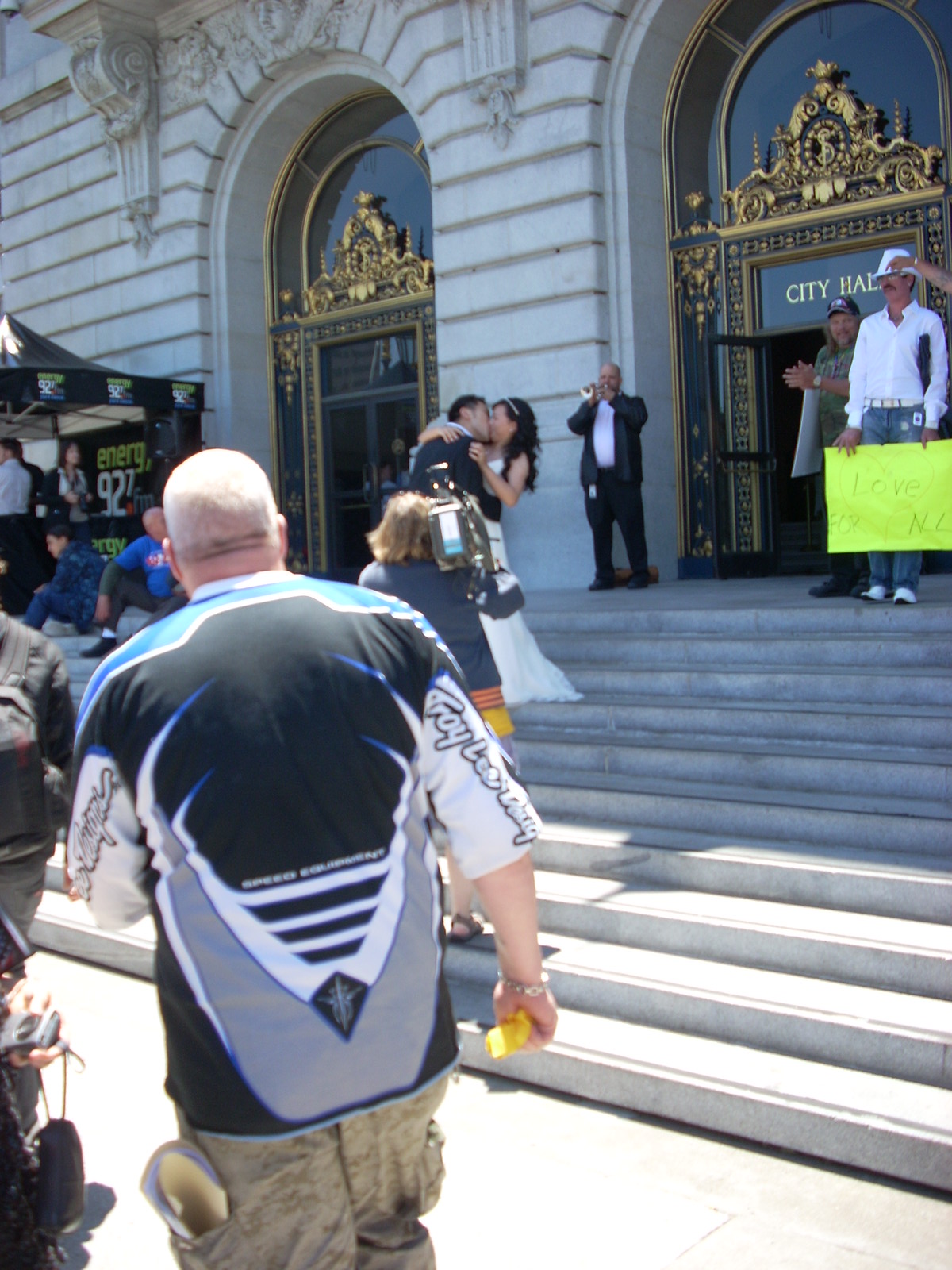In the image, the scene is set outdoors in the middle of the day, in front of an official building marked by a sign that reads "City Hall." The bottom of the frame features a stone brick sidewalk where several people are walking. Leading up to the main doors of City Hall is a staircase, flanked by groups of individuals. Central to the image is a newlywed couple, positioned almost directly in the center, sharing a kiss on the steps. The bride is dressed in a white gown while the groom sports a suit. Behind them, a gentleman with a pronounced paunch wearing a blue suit with a white pullover stands at the top of the steps. Several people around the scene are clapping, and one person on the right is holding an unreadable sign. Others are seated on the steps, seemingly waiting to congratulate the couple. Various colors punctuate the scene, including tan, gray, yellow, blue, black, orange, light green, and gold. In the foreground, to the left, stands a bald, broad-shouldered, broad-hipped man, who appears to be slightly detached from the wedding proceedings.